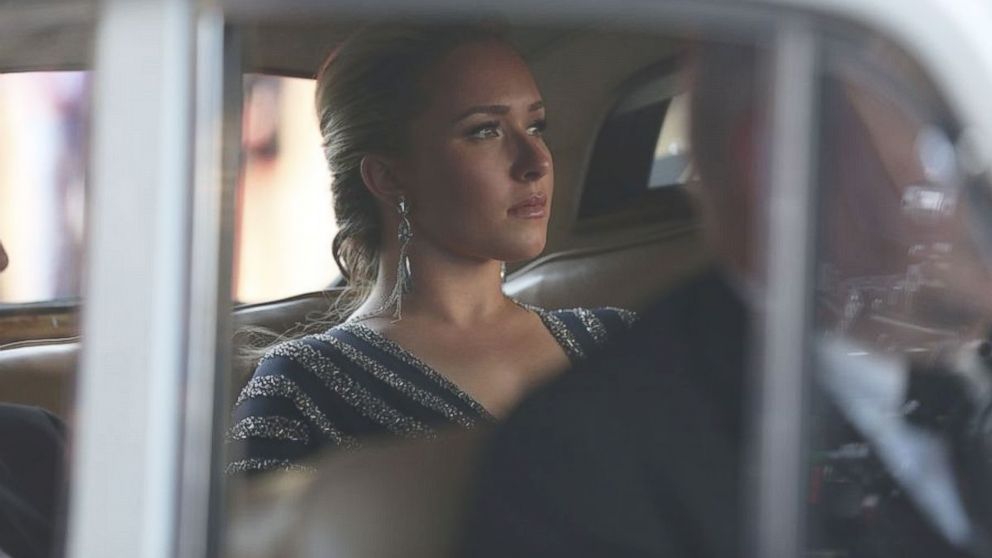In this contemporary image, likely a still from a movie, actress Hayden Panettiere is portrayed sitting in the backseat of a luxurious vehicle, suggesting a limo. The focus is on Hayden, who is elegantly dressed for an evening out; her hair is styled in an updo, accentuating her striking dangling earrings. She is wearing a glamorous, dark blue dress adorned with silver sparkles and jewel-lined fabric. Shifting her gaze to the left, Hayden is framed by the slightly blurry edges of the car window. The backseat is made of brown leather, adding to the luxe atmosphere. In the foreground, the chauffeur, dressed in a black suit, white shirt, and black tie, is partially visible, accentuating the modern sophistication of the scene. The presence of another partially visible figure next to Hayden further enriches the composition, though they remain out of focus, drawing attention to the actress's poised and polished appearance.